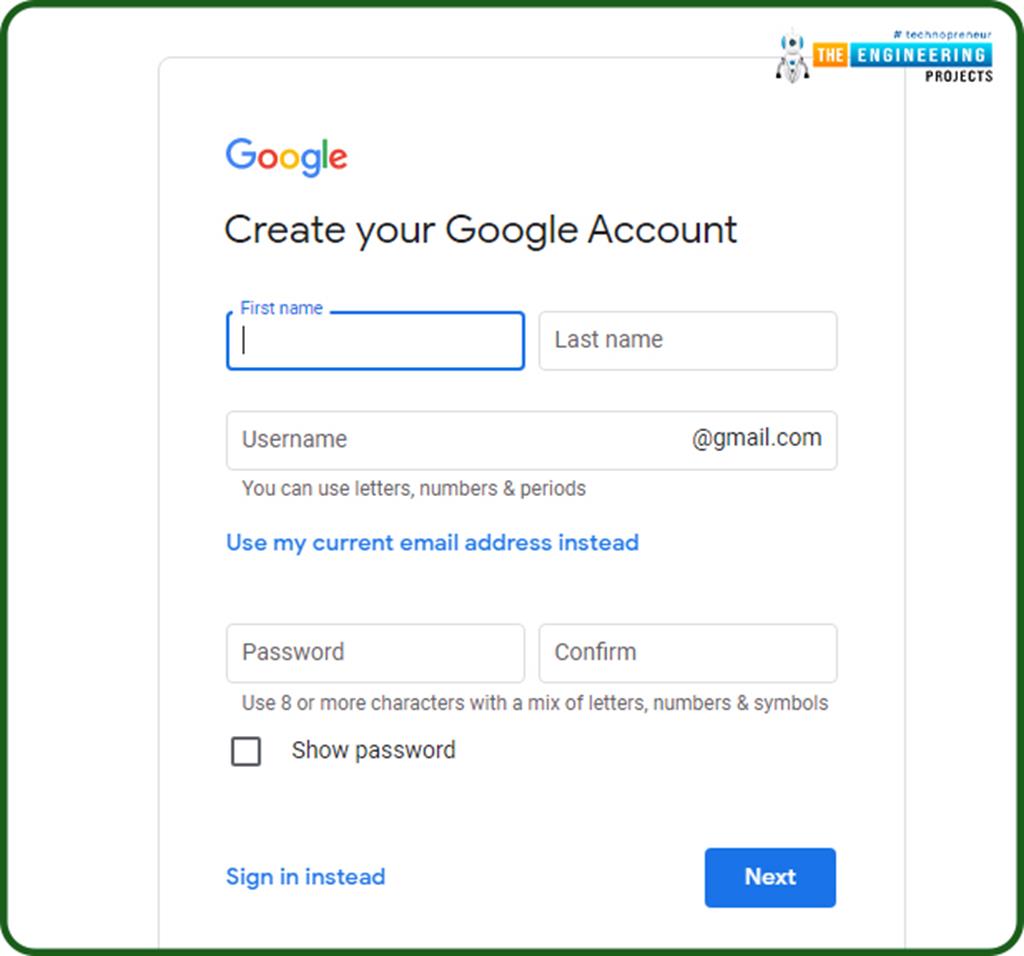The image displays the "Create Your Google Account" menu screen. At the top, the cursor is positioned in the "First name" text box, accompanied by a "Last name" text box to its right. Below these, there is a "Username" text box with an instructional prompt underneath, stating that users can incorporate letters, numbers, and periods in their username. Beneath this prompt is a link in blue text that reads "Use my current email address instead."

Further down, there are two aligned text boxes: the one on the left is labeled "Password" and the one on the right is labeled "Confirm." This section is followed by instructions advising users to create a password using eight or more characters, including a mix of letters, numbers, and symbols. Directly below the password fields is a checkbox option that, when selected, allows the password to be displayed instead of being hidden by black dots.

At the bottom of the menu, there are additional options:
- On the left, a link that says "Sign in instead."
- On the right, a blue rectangular button with the word "Next" written in white text.